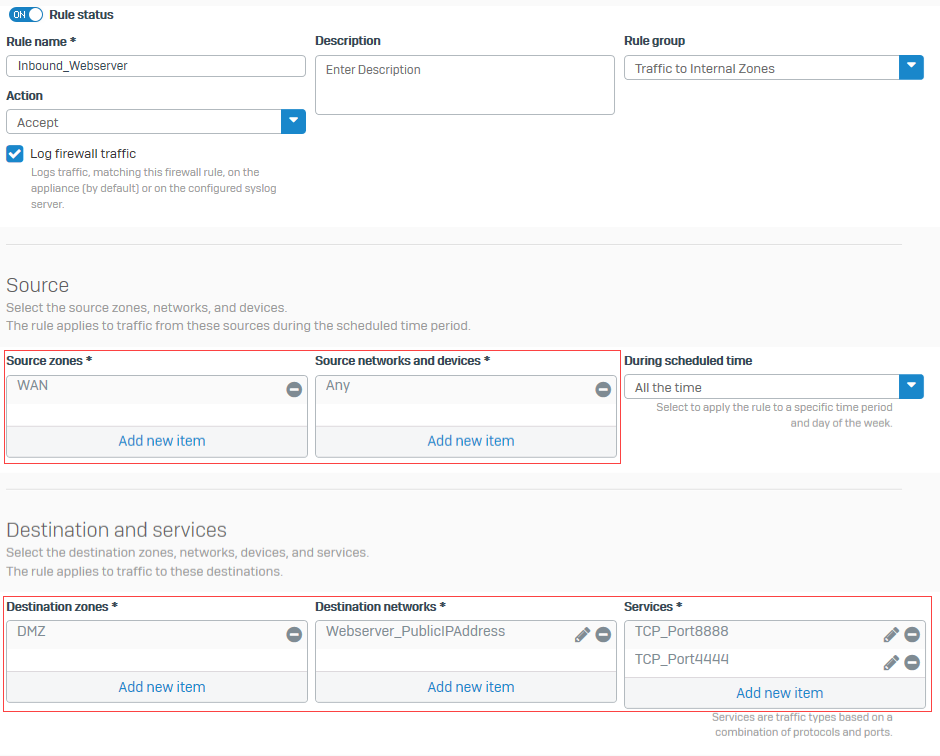This image is a detailed screenshot of firewall settings. At the top left, the screen displays the title "Rule Status." 

The settings consist of several key sections:

1. **Rule Information:**
   - **Rule Name:** Inbound Web Server
   - **Description:** Not provided
   - **Rule Group:** Set Traffic to Internal Zones
   - **Action:** Accept
   - **Log Firewall Traffic:** Enabled, meaning that traffic matching this firewall rule will be logged either on the appliance by default or on a configured syslog server.

2. **Source Configuration:**
   - **Source Zones:** WAN (Wide Area Network)
   - **Source Networks and Devices:** Any (indicating that it applies to all networks and devices within the source zone)
   - **During Scheduled Time:** All the Time (indicating that this rule is always in effect)

3. **Destination and Services Configuration:**
   - **Destination Zones:** DMZ (Demilitarized Zone)
   - **Destination Networks:** Web Server's Public IP Address
   - **Services:**
     - **TCP Port 8888**
     - **TCP Port 4444**
   - **Notes:** Services refer to traffic types defined by a combination of protocols and port numbers.

Overall, the firewall rule detailed in the screenshot allows traffic from any device in the WAN to reach the web server in the DMZ via specified TCP ports, and logs this traffic based on the configured logging settings.